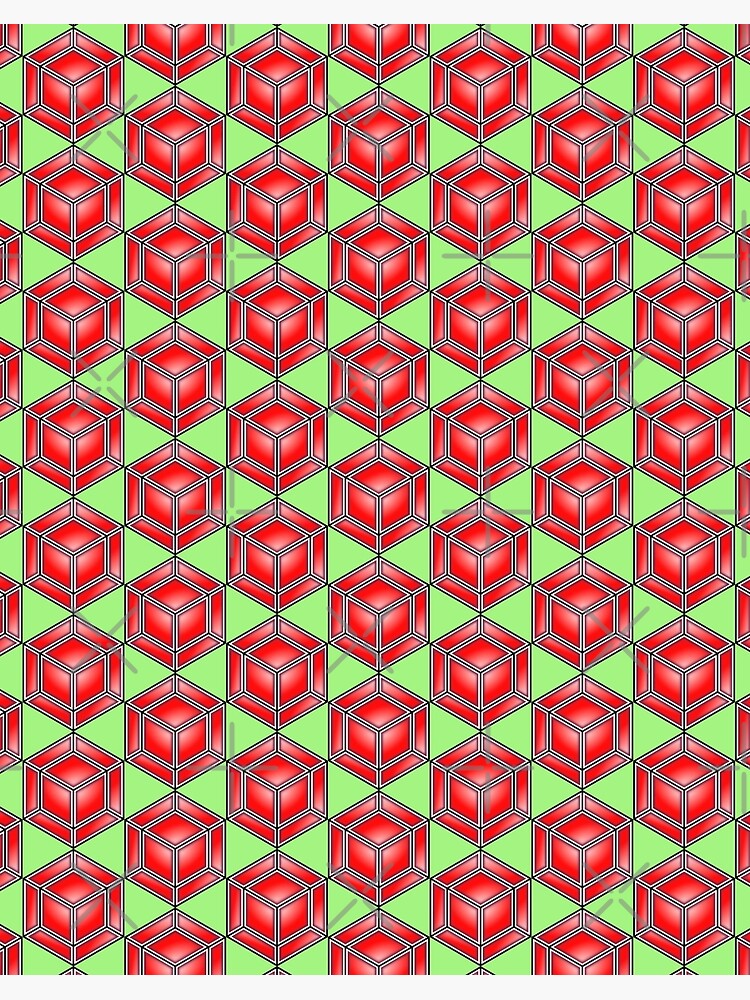This image features a detailed geometric pattern that's ideal for various projects or materials, such as digital artwork, printed paper, or decorative napkins. The central design consists of interlocking squares, each styled in red, and framed with black and white lines, creating the illusion of a cube or a tesseract when viewed from different angles. The background is a refreshing light green, and the pattern is further embellished with subtle light gray watermarks resembling plus and X shapes. Surrounding each square shape is a fine interplay of white, silver, and black accents giving it definition and form. The pattern is organized into seven repeating rows, with continuous elements of red, light green, black, and white throughout, resulting in an intricate and visually captivating design.